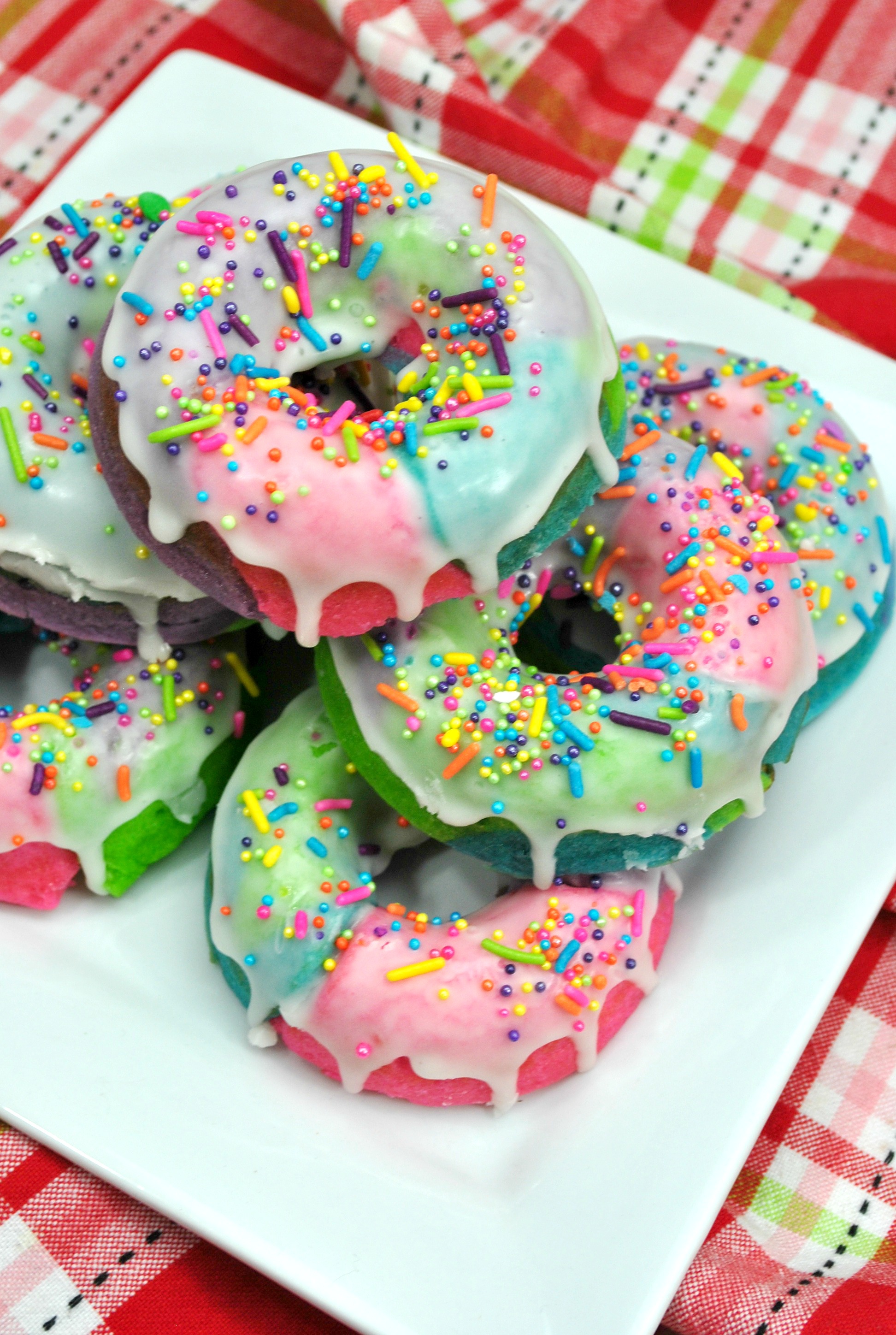This image showcases a visually appealing stack of six to seven donuts arranged in a pyramid formation on a large white square plate. Each donut is uniquely decorated with vibrant colors, including pink, chocolate brown, blue, green, and purple frostings. The frostings are generously coated with an assortment of brightly colored sprinkles in shades of blue, yellow, green, lime, pink, and purple. The sprinkles vary in shapes, ranging from small circles to elongated cones. The icing on the donuts drips slightly over the sides, adding to their homemade charm. The plate sits atop a multi-colored red checkered tablecloth, enhancing the colorful and inviting setting. The overall presentation is clean and neat, making the donuts look even more delectable.